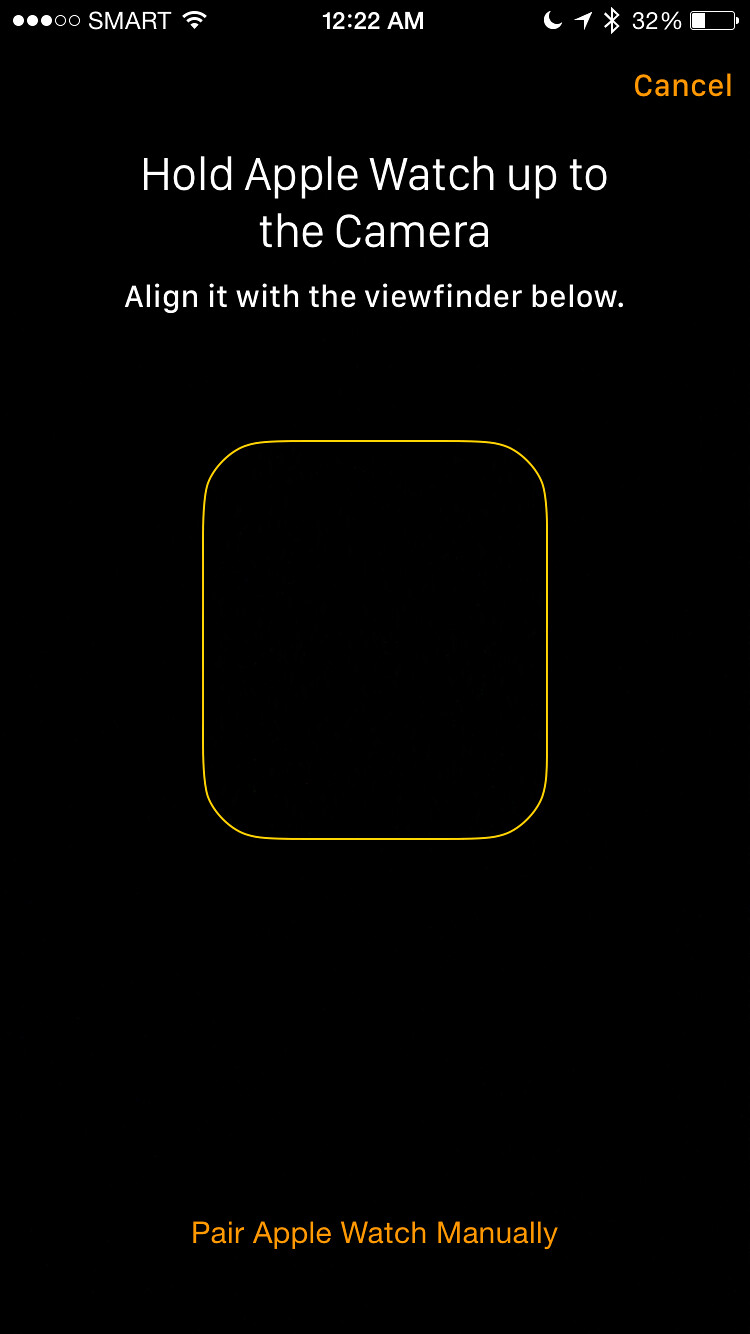The image is a screenshot from an iPhone displaying instructions for pairing an Apple Watch. The backdrop is solid black. At the top of the screen, the status bar shows five dots on the left, with the first three filled in white and the last two outlined but black in the center, followed by the word "SMART" in all capitals. Next to it is a Wi-Fi signal icon. Centrally at the top, the time is displayed as 12:22 a.m. and to the right, there are small icons for a moon, an upward-pointing arrow, Bluetooth, the battery level at 32%, and the battery symbol showing one-third filled. 

Below the status bar, bold white text reads, "Hold the Apple Watch up to the camera" followed by instructions in smaller white text saying, "Align it with the viewfinder below." Centrally in the image is a yellow-outlined rounded square, which serves as the viewfinder. At the bottom, there is an orange text option, "Pair Apple Watch Manually."